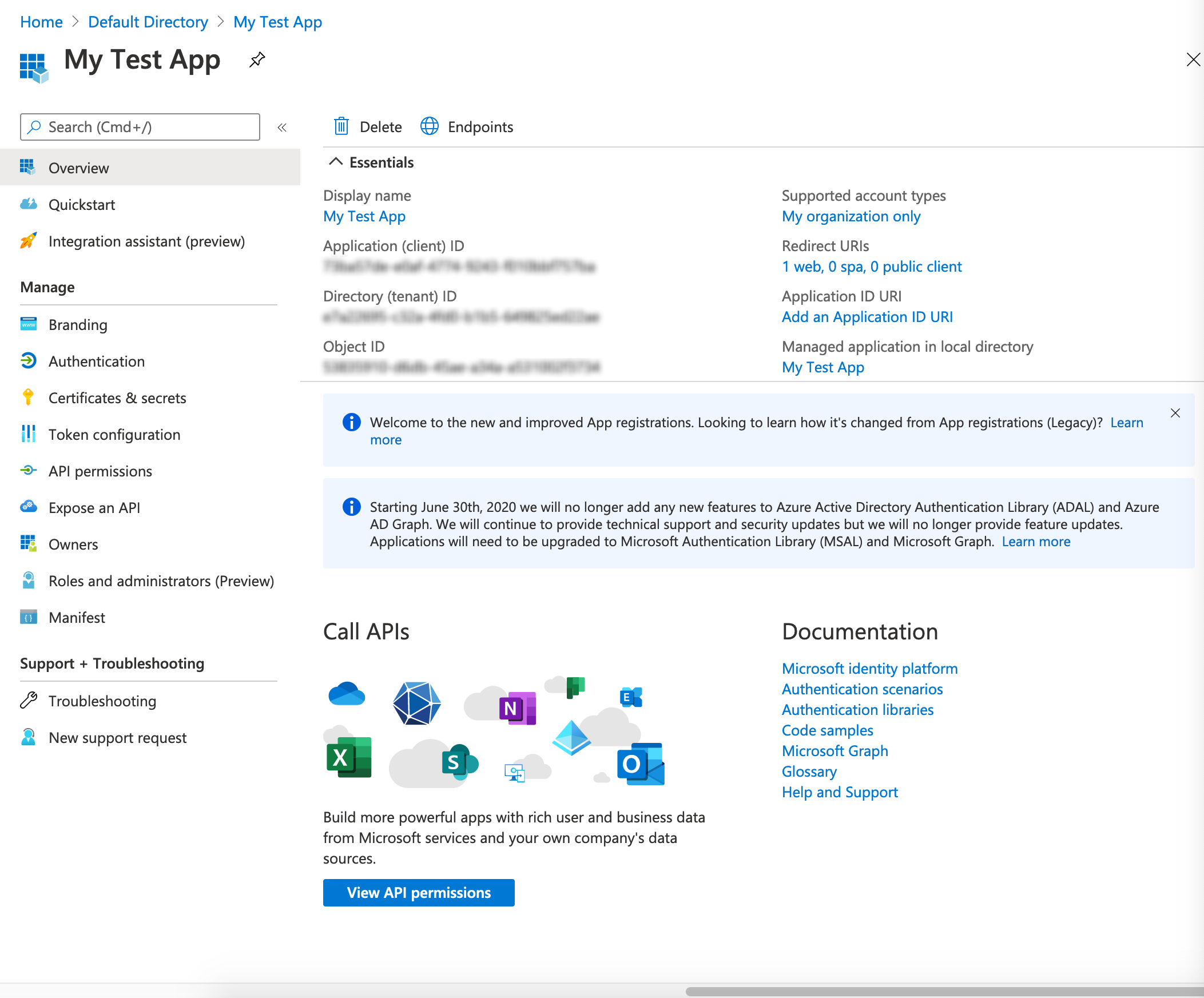The image is a detailed screenshot of a possible laptop or tablet interface, showcasing a developer's application dashboard. At the top, the word "Home" is displayed in blue, accompanied by an arrow pointing to the "Default Directory" and another arrow indicating "My Test App." Below this, a square icon containing smaller squares, and a cube positioned outside it is visible, representing the test application. 

A thumbtack icon also appears, pointing to the side. Directly underneath, a search bar with a magnifying glass icon is labeled "Search," and on the opposite side, there is an icon of a trash can labeled "Delete."

In the section titled "Endpoints," an icon resembling the Earth is present. Below this, the heading "Essentials" is followed by various subtopics including "Display Name." On the left panel, "Overview" is highlighted, with "Quick Start Integration" listed underneath, accompanied by a rocket icon.

Further down, "Manage" displays subgroups such as "Branding," "Authentication," "Certificates," and "Secrets," each with their respective small icons. A blue exclamation mark highlights an important area, which contains two faded rectangles with additional information.

At the bottom, the section labeled "Call APIs" includes a highlighted "View API Permissions" button. On the right-hand side, there is a "Documentation" section featuring multiple subheadings.